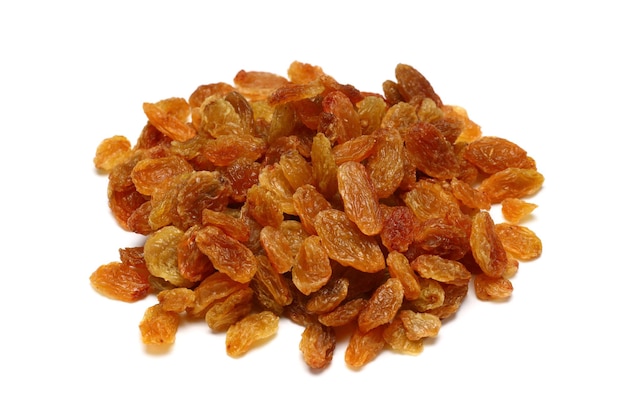This is a highly detailed photograph of a pile of golden raisins, with a clean, white, translucent background. The raisins are piled together without any visible borders, emphasizing their uniformity in size and shape. The colors of the raisins vary slightly, each having their own unique hue, ranging from a very light yellow to a copperish, reddish-orange. Some of the raisins exhibit a rust-like color, and the array of shades includes light orange and darker brown tones. The raisins appear very dry and wrinkly, indicative of dehydration, as if they were left out in the sun. This bright and well-lit image showcases the nuanced texture and varied coloration of the raisins, revealing some lighter off-white spots on certain pieces, suggesting a mix of green or golden grapes at different stages of dehydration.